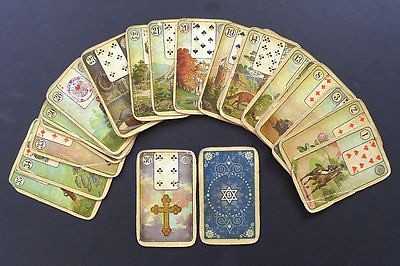On a dark purple background, an assortment of ancient, intricately textured playing cards is spread across the table in a loose, U-shaped arrangement. Among the cards, the one on the left stands out with its Christian-themed imagery, while the card on the right is distinctly blue. The cards numbered 1, 2, 3, 8, 13, and 14 exhibit a different design, further emphasizing the historical and eclectic nature of the collection. The overall composition displays the cards in various orientations, creating a dynamic and engaging visual scene.